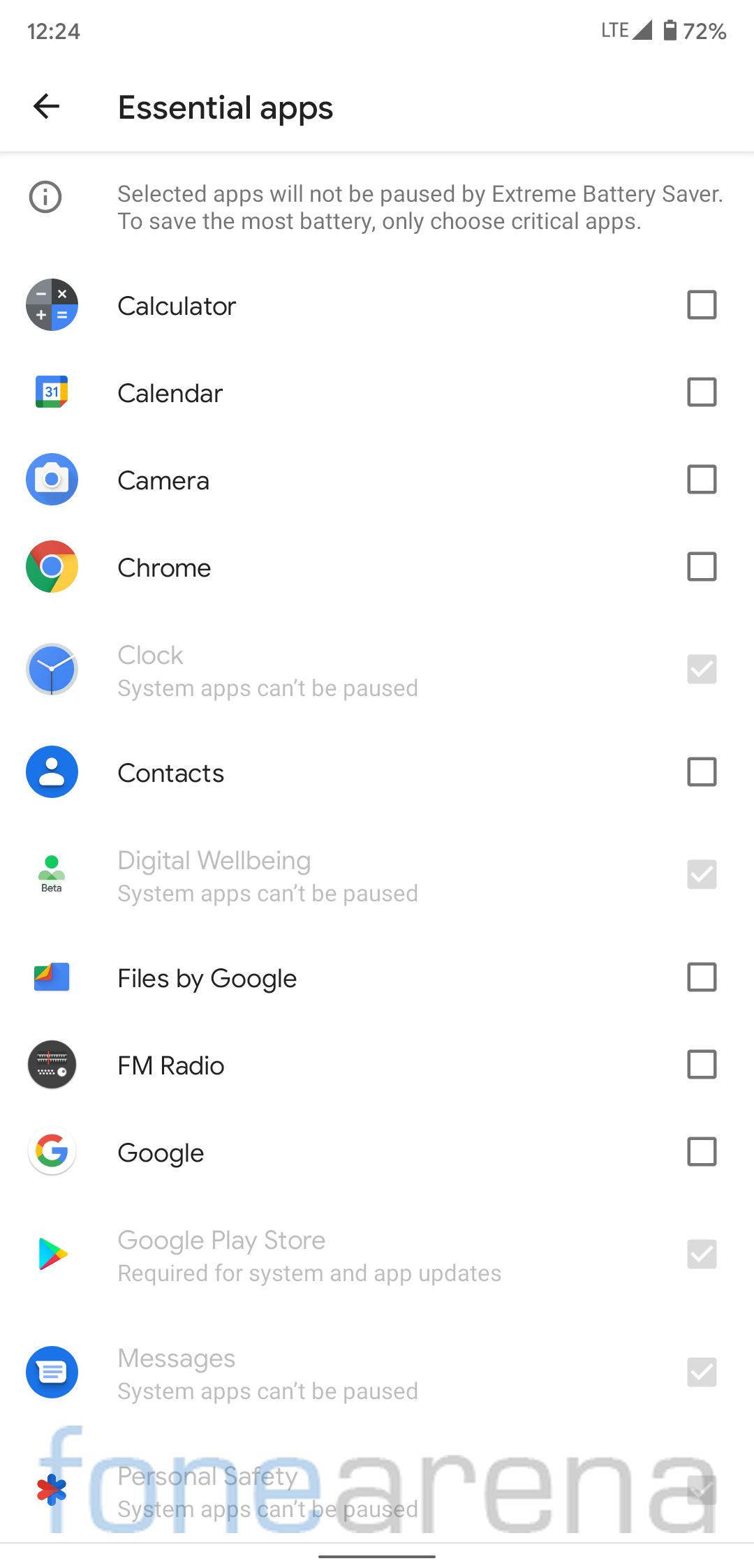The screenshot depicts the "Essential Apps" page from a mobile device, captured on a clean, white background with ample empty space. The device's interface shows the time as 12:24 in the upper left corner, with various status icons, including a battery indicator displaying 72% charge, situated in the upper right corner. The top navigation bar features the title "Essential Apps" alongside a left-pointing arrow icon, indicating a navigation option to return to the previous screen.

Directly below, a single vertical line divides the screen, providing a subtle separation of content. The page exhibits a mixture of grayed-out areas and interactive elements. Along the right side, there are multiple checkboxes—some marked while others remain blank—aligning with a list of categorized apps.

Among the unchecked categories are:
- Calculator
- Calendar
- Camera
- Chrome
- Contacts
- Files by Google
- FM Radio
- Google

The checked categories appear in light gray and include annotations "System Apps Can't Be Paused" or "Required for System and App Updates":
- Clock
- Digital Well-Being
- Google Play Store
- Messages
- Personal Safety
  
At the bottom of the image, the watermark "FONEARENA" is clearly visible, solidifying the source of the capture. Overall, the image’s minimalistic white background complements the textual content, keeping the focus on the interface details.